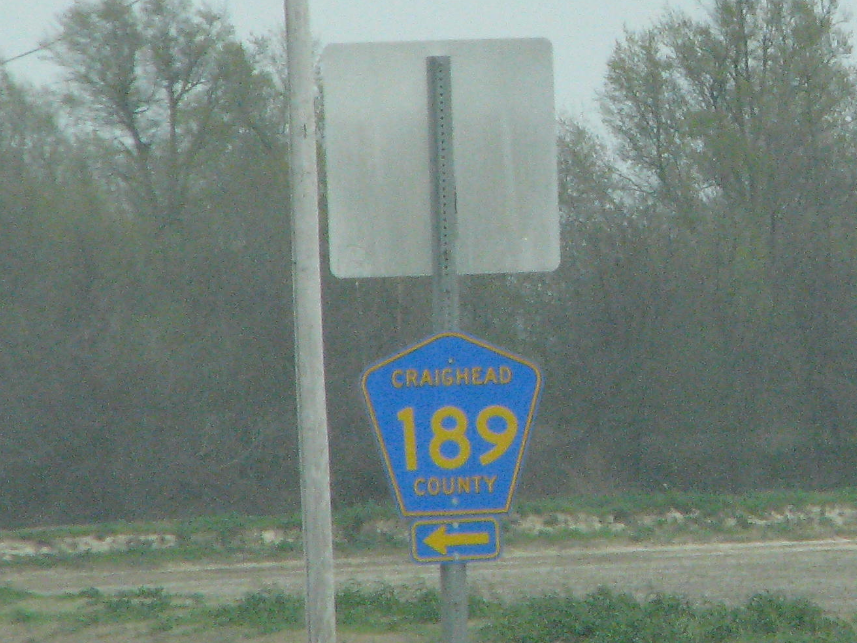This is a close-up photograph of a county road sign on the side of a road in Craighead County, identified as Route 189. The sign features a blue background with a yellow border and displays "Craighead" in yellow letters at the top, "189" in large yellow font in the center, and "County" in smaller yellow font beneath the number. Below this main sign is a smaller blue rectangular sign with a yellow left-pointing arrow. These signs are mounted on a steel pole. Above the main sign, there's another sign facing the opposite direction, likely a "Do Not Enter" or "Wrong Way" sign, visible only from the back with white and gray coloring. To the left of the pole is an old, weathered wooden utility pole, now grayish in color. The scene includes a road running horizontally at the bottom of the image, with sparse grass along its edges and a dense forest of deciduous trees, their green leaves creating a lush backdrop. The photograph is of grainy quality, adding a nostalgic feel to the otherwise vibrant setting.